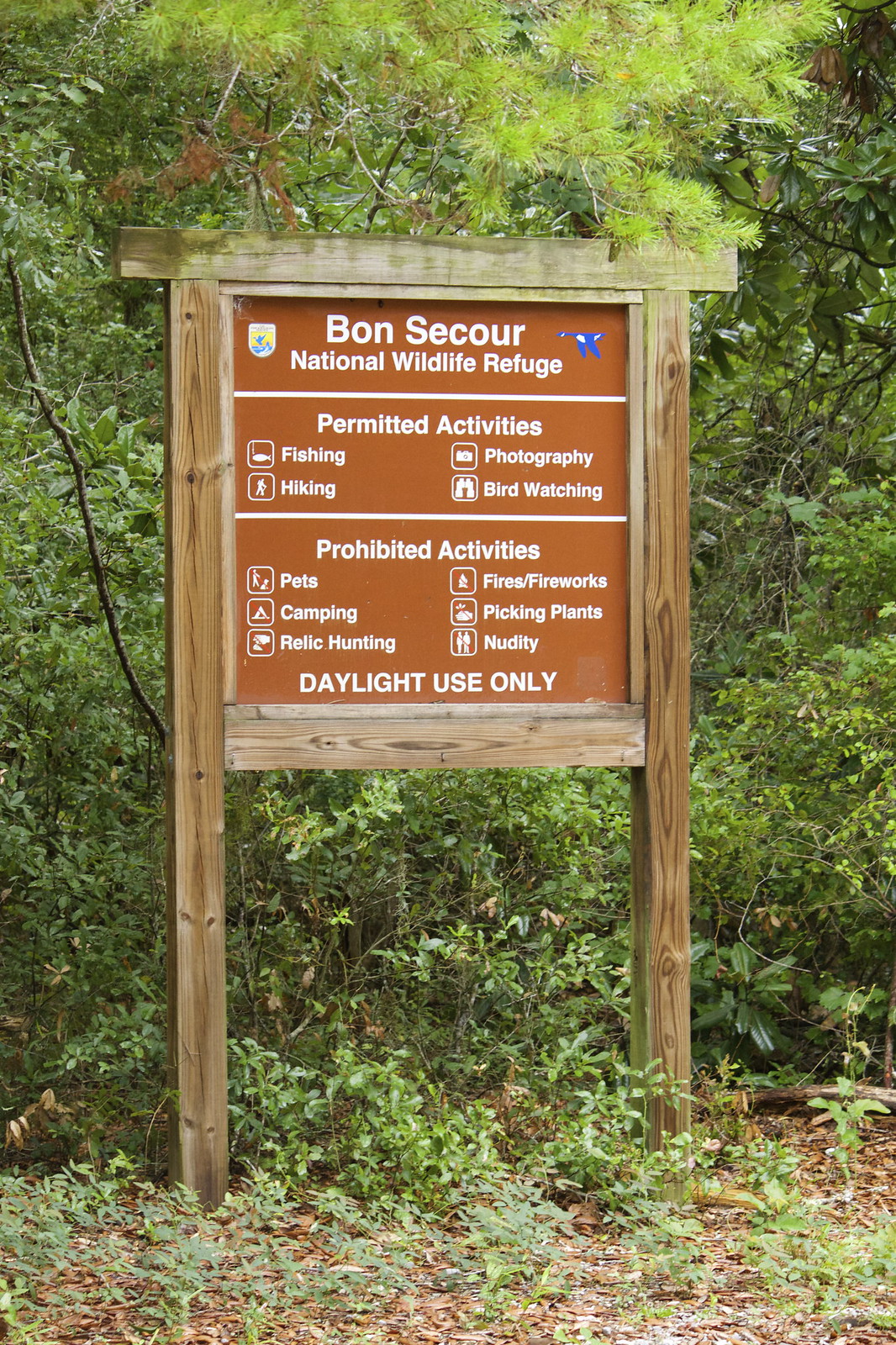This full-color vertical photograph, taken on a sunny day in the woods, captures a distinctive rustic scene typical of a national park setting. Dense trees with a mix of bright green and darker foliage form the backdrop, while the ground is an earthy mixture of dirt, mulch, and weeds. 

At the center, prominently displayed, is a brown wooden sign mounted on two vertical wooden posts, enhancing its presence against the natural backdrop. The sign is framed by additional horizontal wooden supports at the top and bottom, forming a sturdy square frame.

The sign, with its solid medium-brown background and crisp white text, reads "Bon Secours National Wildlife Refuge" at the top, above a white horizontal line. The next section lists permitted activities – fishing, hiking, photography, and bird watching – each illustrated with small icons. Another white horizontal line separates this from the section below, which outlines prohibited activities including pets, camping, relic hunting, fireworks, picking plants, and nudity, each paired with icons crossed out with a red strikethrough. Emphasizing the rules, the bottom of the sign declares in bold, all-caps white letters: "DAYLIGHT USE ONLY."

Additional embellishments include a badge-like crest image on the left and a blue bird icon on the right, lending an official and inviting character to the sign. The detailed directives paint a clear picture of the park's expectations, ensuring that visitors enjoy the Bon Secours National Wildlife Refuge responsibly and respectfully.